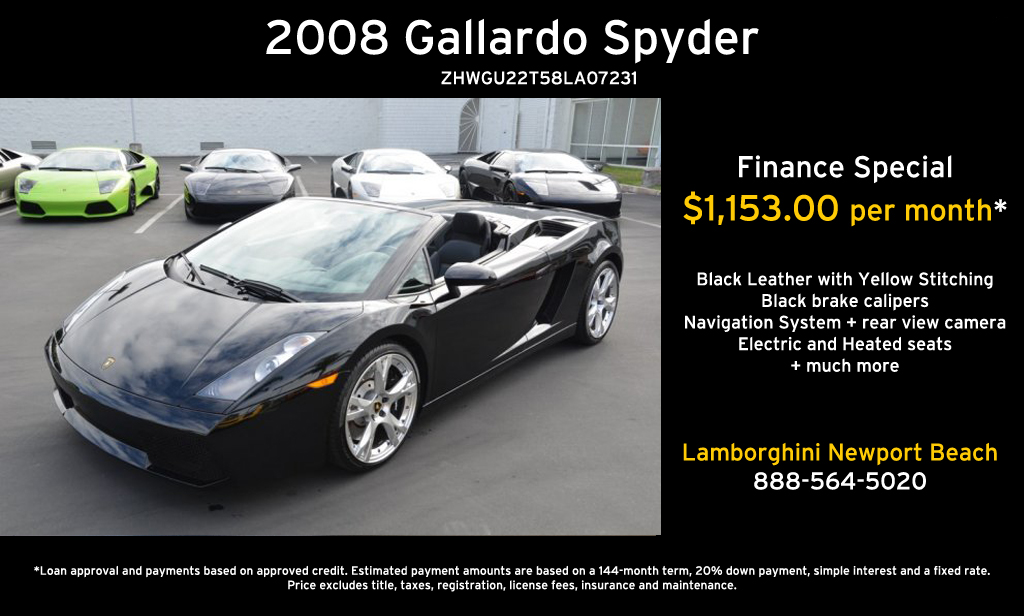This advertisement showcases a 2008 Gallardo Spyder, prominently featuring the car in a sleek landscape-oriented color photograph. The car is a black, two-seat convertible, with its sunroof down, positioned at an angle facing the bottom left corner. It stands out against a backdrop of four other cars in green, black, white, and silver, parked on a concrete lot with a white building behind them. The focus remains firmly on the 2008 model, its shiny wheels and black brake calipers adding to its allure. 

Above the image, in bold white sans serif font, the headline reads "2008 Gallardo Spyder," with additional small lettering providing an ID number. To the right, the text "Finance Special" is displayed, followed by "$1,153 per month" in gold lettering, and a list of features including black leather seats with yellow stitching, a navigation system, rear view camera, and electric heated seats. Below this, the text "Lamborghini Newport Beach" appears in yellow, accompanied by the contact number 858-564-5020. At the bottom edge, a disclaimer in small white text explains that loan approval and monthly payments are based on approved credit, with terms including a 144-month duration, 20% down payment, simple interest, and a fixed rate. Additional costs like title, taxes, registration, license fees, insurance, and maintenance are excluded. The advertisement masterfully blends photographic realism with graphic design typography against a solid black background.